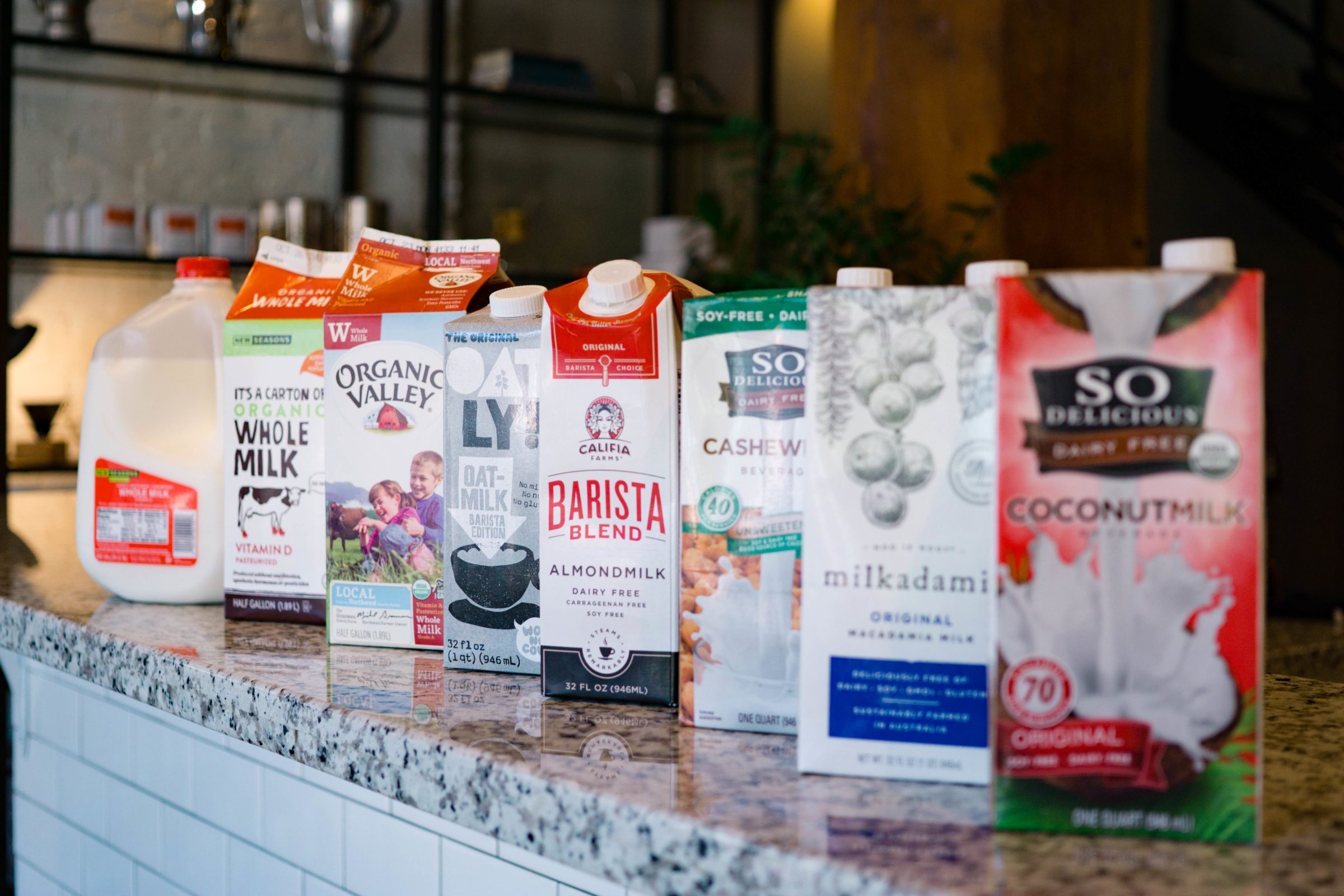This photograph showcases an assortment of eight different types of milk arranged on a granite countertop with white tile beneath it, set against the blurry backdrop of what appears to be a coffee shop with shelves, a plant, and a wooden beam in the background. From left to right, the milks are:

1. **Regular Whole Milk**: A gallon jug featuring a red label and red topper, though the text is not legible.
2. **Organic Whole Milk Vitamin D**: A half-gallon carton with an orange top, sporting a photo of a cow and labeled as organic.
3. **Organic Valley**: Another half-gallon carton with an orange top, adorned with a W and depicting a young boy and girl playing in a field with a cow in the background.
4. **Oatly Barista Edition**: An oat milk in a 32-ounce gray carton with a white topper, specifically labeled for barista use.
5. **Califia Farms Barista Blend Almond Milk**: This dairy-free option comes in a primarily white carton with red and black accents and a white screw top.
6. **So Delicious Cashew Milk**: A green and white carton marked as soy-free and dairy-free, featuring an image of milk pouring into a glass with almonds in the background.
7. **Milkadamia Original**: Housed in a white carton with blue and green accents, it features illustrations of macadamia nuts.
8. **So Delicious Coconut Milk**: A red and white carton with green accents, depicting milk pouring into a coconut, also marked as dairy-free.

These diverse milk options highlight the range of dairy and plant-based milks available, set against the bustling ambiance of a coffee shop.